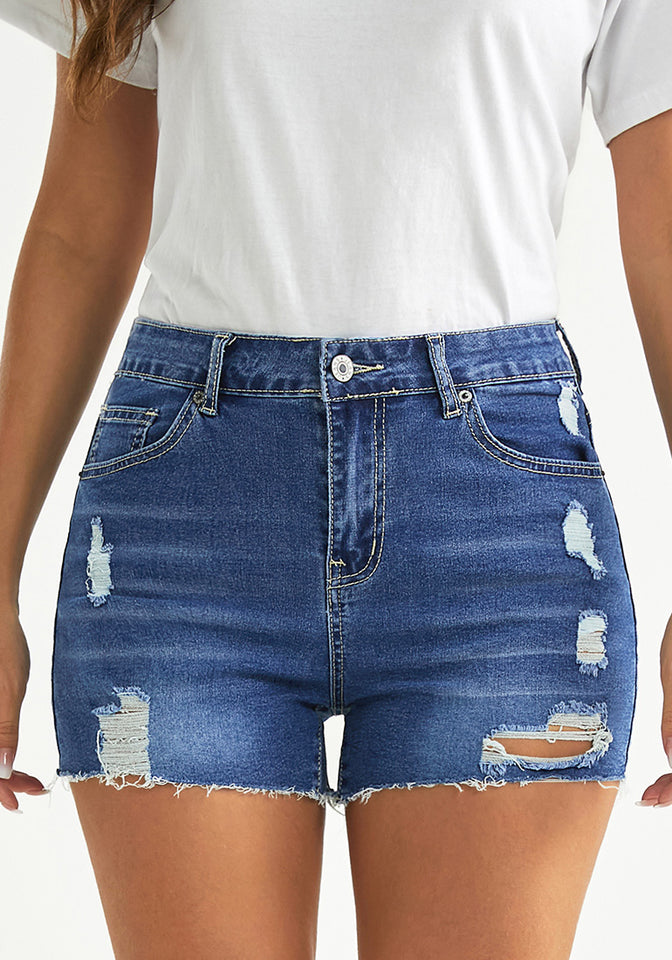This vertically-aligned, rectangular photograph showcases a woman, captured from mid-chest to just above her knees. She is wearing a white half-sleeve T-shirt tucked into blue denim cut-off shorts that are fashionably distressed with intentional rips, displaying white threads beneath. The shorts, secured with a round button and zipper, feature two side pockets and an additional mini pocket on the left. The clearly visible rips are more pronounced on the right side, with the left side showing only a couple. Both of her arms hang naturally by her sides, revealing a French manicure on one visible nail. At the top left corner, a wisp of her long, brunette hair falls past her sleeve. The background is a plain, solid white, emphasizing the focus on her casual yet stylish outfit.